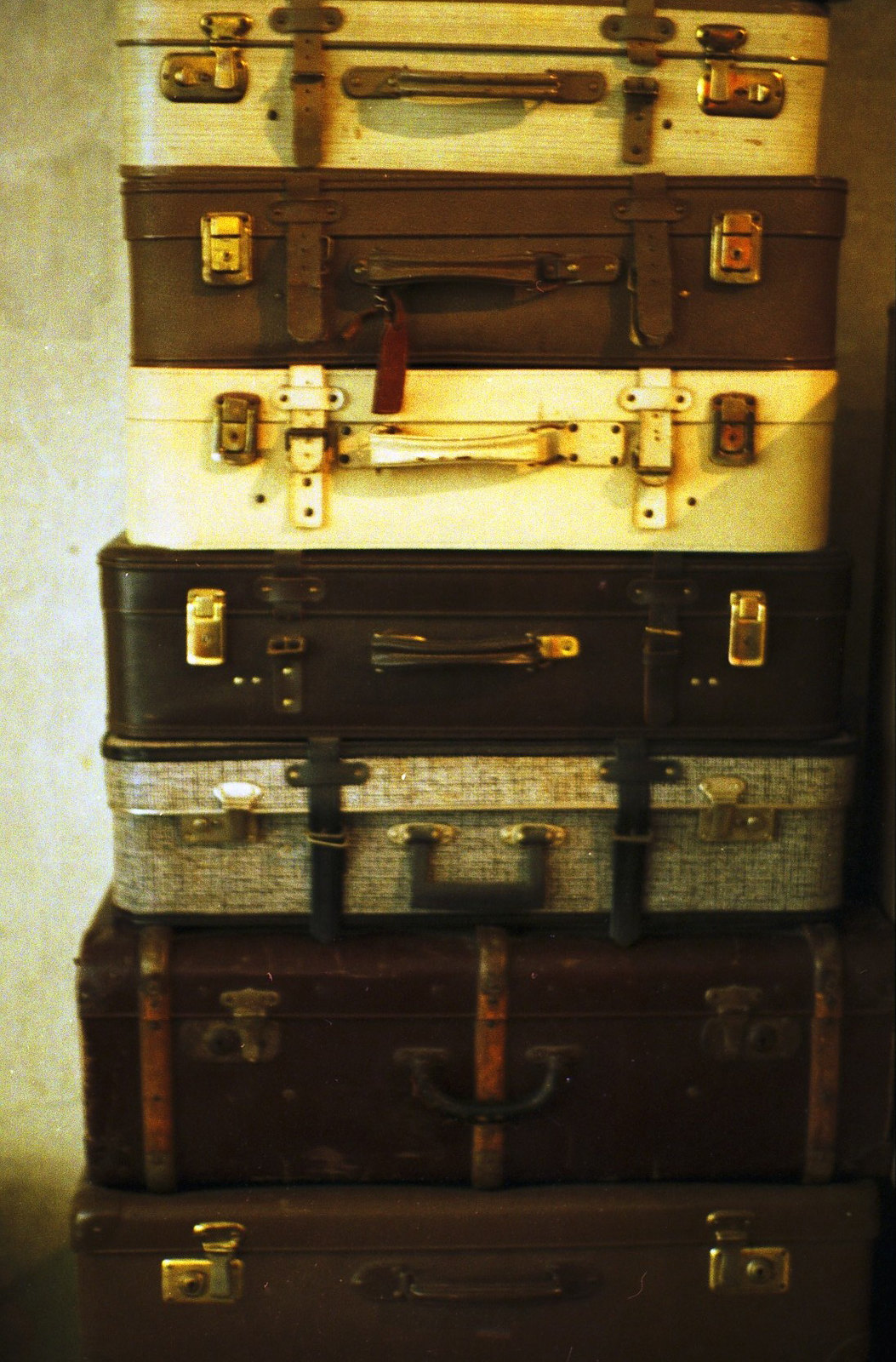This detailed photograph, with a somewhat blurred and yellowish filter, captures a tightly cropped view of a tower of seven vintage suitcases stacked horizontally. The suitcases, filling the entire frame, range in color and style, creating a visually intriguing pattern. Starting from the bottom, the base is a medium-brown steamer trunk reminiscent of the early 1900s, followed by a darker brown suitcase. Above it is a suitcase featuring an off-white and black crisscross woven design. Continuing up, a black leather suitcase with classical buckles and flaps rests beneath a predominantly white suitcase accented with brown leather buckles. Near the top is another brown leather suitcase, potentially adorned with brass buckles. Crowning the stack is a white suitcase, slightly dirtied from extensive use. Golden buckles and visible handles punctuate the design of each piece. The image also hints at an indoor setting, with a slight view of what might be a wall on the left side. There are no texts or signatures visible in the photograph.